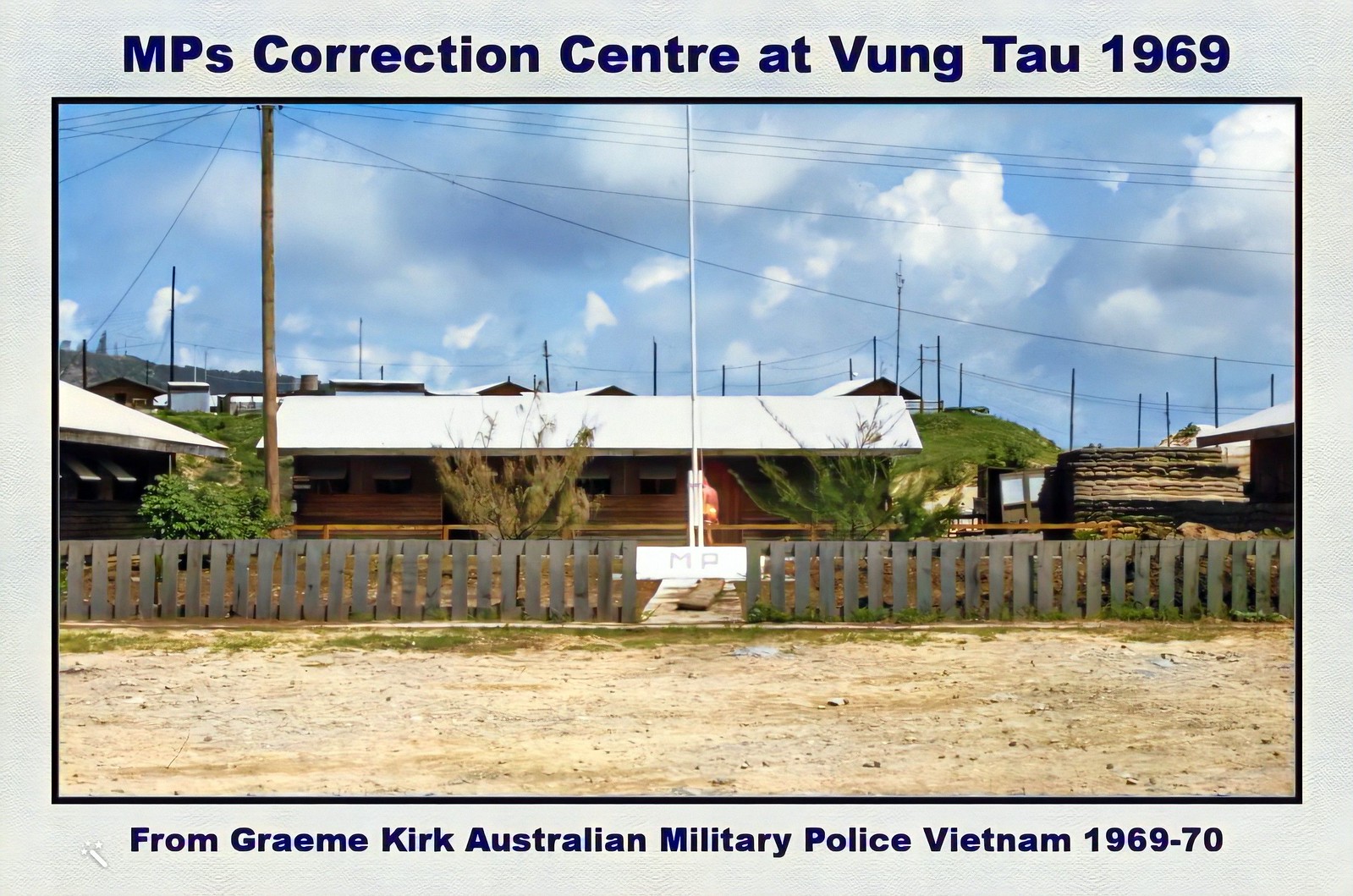This historical photograph from 1969 is centered around the MP's Correction Center at Vung Tau during the Vietnam War, and it comes with the annotation "from Graeme Kirk, Australian Military Police, Vietnam 1969-70." The image is framed by a light blue background with bold dark blue text at the top and bottom, specifying its historical context. The photograph itself is in the middle, bordered by a black frame.

In the foreground, a dirt and gravel lot is dotted with patches of grass, leading up to a short wooden picket fence with a central walkway. A white sign with the large gray letters "MP" is affixed to the fence. Beyond the fence, there is a one-story reddish-brown building with a white rooftop and small windows, likely serving as the correction center mentioned. To the right of this building is a large, stone or brick structure.

The background includes rolling grassy hills and a collection of telephone poles and wires stretching across a partly cloudy, brilliant blue sky. A flagpole can be seen, behind which a single person appears, mostly obscured. The combination of these elements paints a detailed picture of the correctional center's environment amidst the tumult of the Vietnam War.